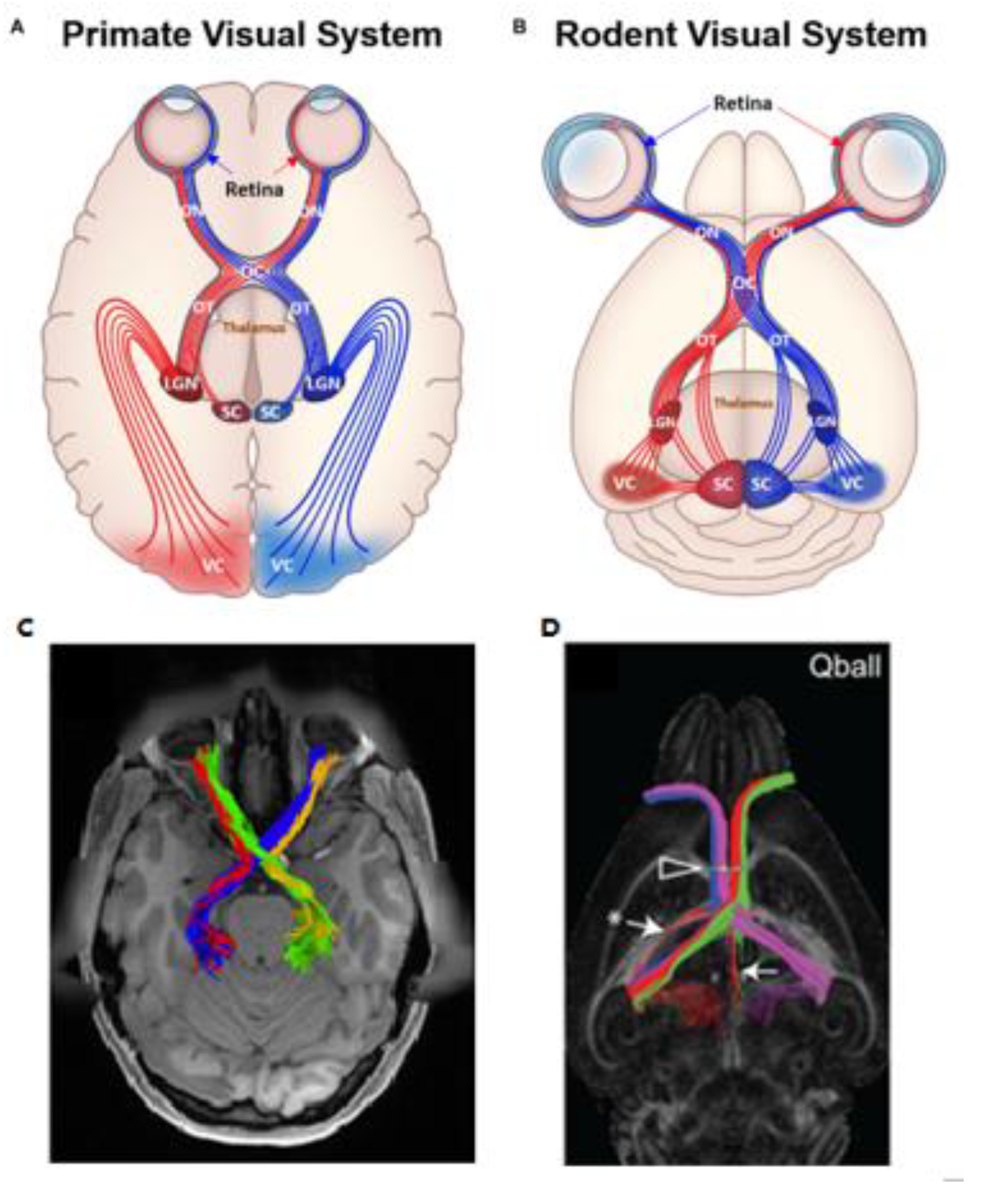The image depicts a comparative analysis of the visual systems in primates and rodents, presented in a detailed, four-part illustration. The top of the illustration features two schematic diagrams labeled A and B, showcasing the visual systems of primates and rodents, respectively. The primate visual system is illustrated with a pink brain, red and blue lines representing potential arteries and veins, connecting the retina and eyes at the top to various parts of the brain. Similarly, the rodent visual system diagram shows a beige outline of the rodent brain with analogous blue and red lines extending from the eyes to the brain, though with differences in pathway structures compared to the primate system.

The bottom section includes two images labeled C and D, which appear to be x-rays or scans of the actual brains. Image C represents the human or primate visual system, featuring colored lines in red, green, blue, and yellow that trace neural pathways from the eyes to the brain. Image D illustrates the rodent visual system with similar multicolored lines in pink, blue, green, and red, but arranged differently, reflecting variations in the rodent's neural pathways. The overall setup combines schematic and realistic depictions, offering both a high-level and detailed view of visual system structures and connections in these animals.